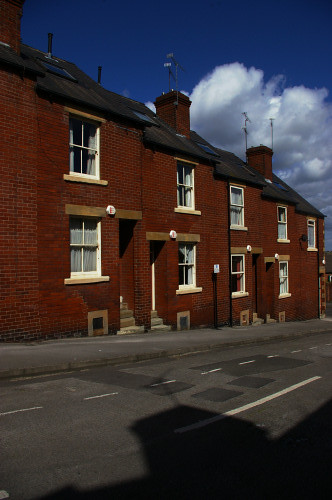The image showcases a bright blue sky with a large white cloud in the top right corner. Below, a street runs diagonally from the bottom left to the middle right of the frame. On the left side of the street, there is a series of attached brown and red brick buildings, each with two floors. Every building features a window and a door on each floor, complemented by windows with white panels. Atop each building is a black roof with a chimney and some have a sunlight window. The entrances to the buildings are accessible via small concrete steps. 

Running parallel to these buildings is a concrete sidewalk, and the street itself features both solid and dotted white lines in the middle. Additionally, there are separate white lines near the curb of the sidewalk adjacent to the houses. The detailed architectural elements and road markings give the scene a structured yet inviting appearance.